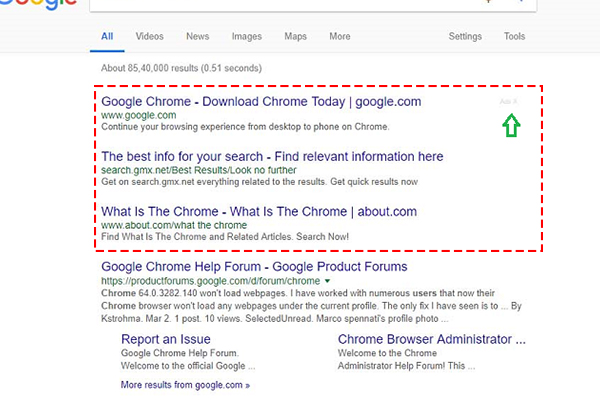This image captures a screenshot from a Google search results page. The Google logo is partially visible, with only the bottom third discernible, along with the search bar. Below the search bar, the different categories of search results are listed, such as "All," "Videos," "News," "Images," "Maps," and "More," with the "All" category highlighted.

The page indicates that approximately 85 million results were found. The top three search results are encapsulated within a red dashed-bordered rectangle, distinguishing them from the rest. These highlighted results include:
1. "Google Chrome - Download Google" 
2. "Google.com - The Best Info for Your Search - Find Relevant Information Here"
3. "What is Chrome? - About.com"

Beneath this highlighted section is another, singular result: "Google Chrome Help Forum - Google Product Forums." The detailed layout provides a clear visual hierarchy of the search results, emphasizing the most relevant links at the top of the list.